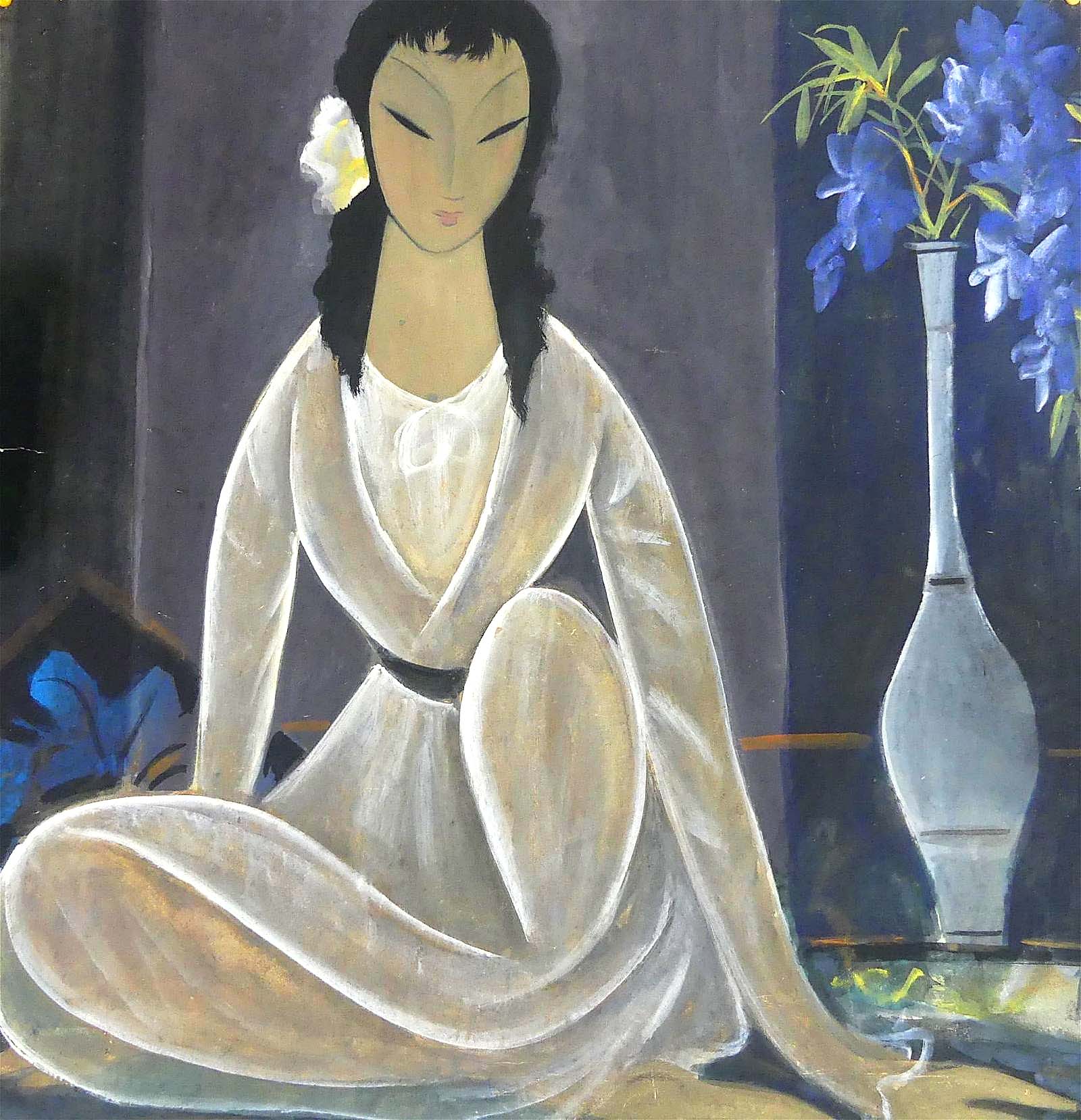The painting features an Asian woman sitting on the ground, with one knee drawn up to her chest and the other leg out to the side. She has long black hair adorned with a white flower and is dressed in a white robe with a black belt around her waist. Her eyes are small, slanted, and appear closed. The background includes a gray column, giving a sense of structure, while the right side of the image has dark tones suggesting a nighttime ambiance. To her right stands a tall, white vase with an exceptionally elongated neck, holding blue flowers and greenery. To the woman's left, partly obscured behind her, appears to be a black diamond-shaped object featuring a blue flower pattern, possibly a pillow. The painting employs a palette of white, blue, and gray hues, creating a cold and serene atmosphere.